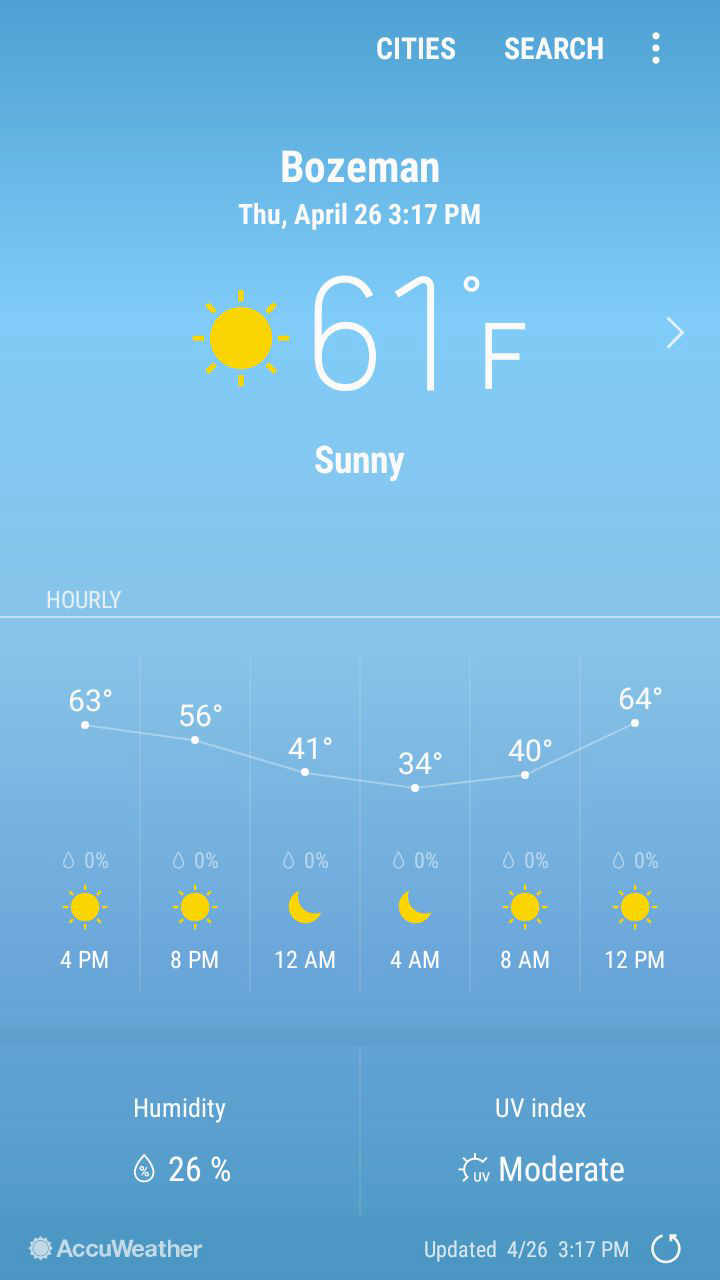Here is a detailed and cleaned-up version of the caption for the image:

---

This image is a screenshot from a mobile weather app featuring a clear blue background. In the upper left corner, white text reads "Cities" with a "Search" field immediately below it. Beneath these, there are three vertical white dots indicating additional options. The main display shows the city name "Bozeman" at the top, followed by the current date and time: "Thursday, April 26th, 3:17 PM." Below this, a sun icon—an orange circle with radiating orange dashes—indicates sunny weather. To the right, large white text displays the current temperature: "61°F," accompanied by a small arrow pointing to the right. Under this information, the text "Sunny" is indicated. 

In the lower right corner, a label "Hourly" is displayed with a thin white line beneath it. Below, a chart showcases the hourly weather forecast starting at 4 PM and continuing until 12 PM, predicting temperatures ranging from 63°F to 64°F, with all listed hours showing 0% humidity. 

At the bottom of the screen, in the lower left, the text "Humidity: 26%" appears, and in the lower right, the UV index is labeled as "Moderate." The image is concluded with the "AccuWeather" logo at the very bottom.

---